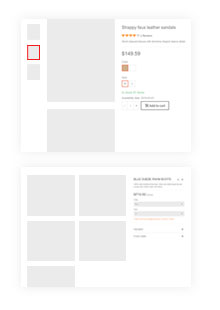The image depicts a blurry screen, which is visually confusing and lacks clarity. At the top of the screen, three smaller blue rectangles are aligned vertically on the left side, adjacent to a large central blurred rectangle. The middle of the three smaller rectangles is highlighted in red, suggesting it might be linked to a product, inferred by a faint indication of a price. Below this section, the lower half of the screen features four equal-sized blue rectangles positioned side by side horizontally, with some text appearing to their right. Additionally, a smaller horizontal rectangle is located at the very bottom. Despite the detailed layout, the content remains indecipherable due to the pervasive blurriness, making it impossible to identify the specifics of the page.